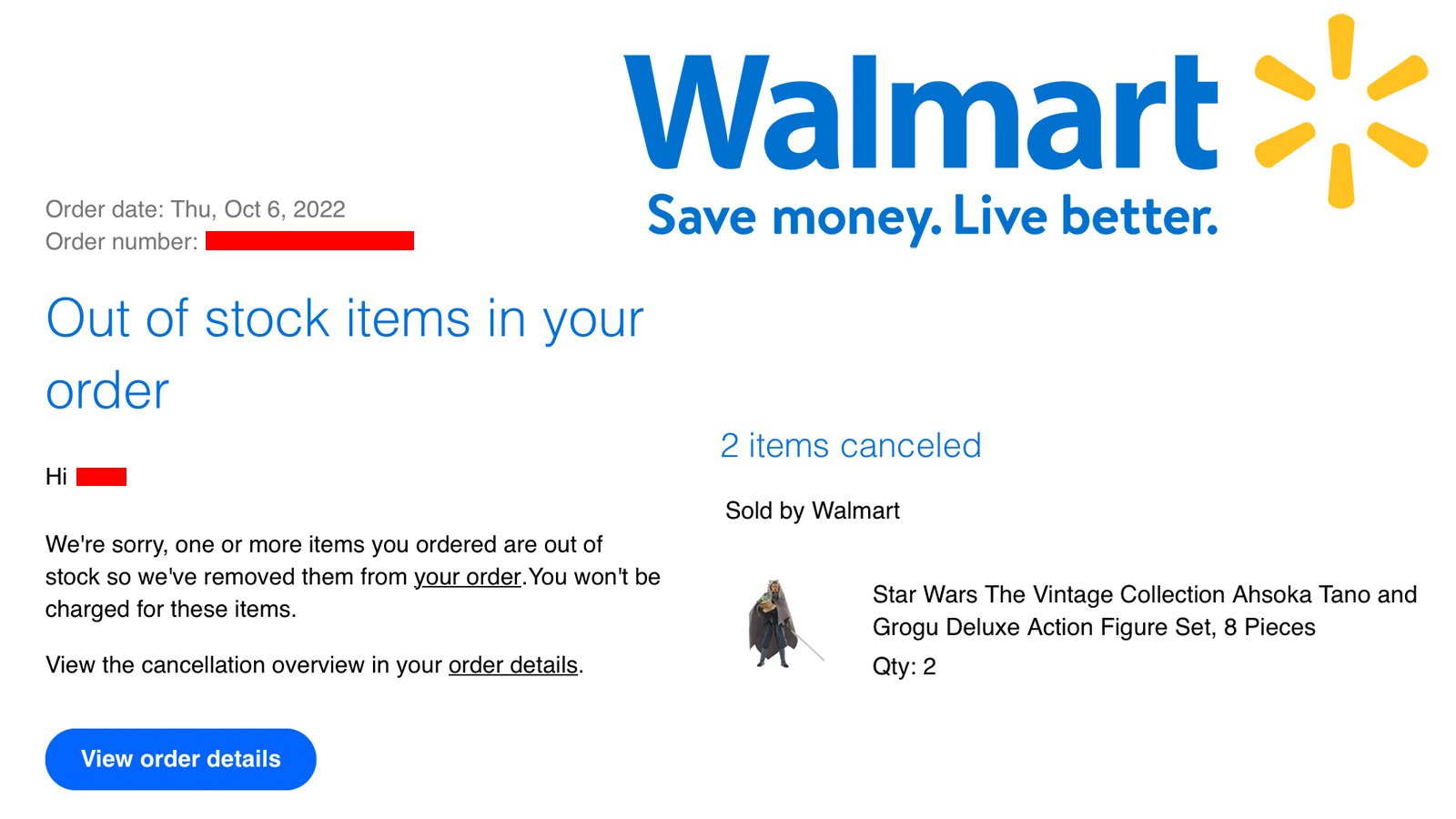The image features a two-column notification with a white background. 

**Left Column:**
- At the top, in black text, it reads "Order Date" followed by a colon, and then "THU, October 6th, November 2022."
- Beneath the Order Date, it says "Order Number: [...]", but the order number is redacted and not visible.
- In blue text, it states "Out of Stock Items in Your Order," followed by "Hi," which is also redacted.
- A message in black text follows, "We're sorry, one or more of the items you ordered are out of stock, so we removed them from your order." The phrase "your order" is underlined.
- It continues, "You won't be charged for these items due to cancellation." The phrase "Order Details" is underlined.
- There is a blue underline beneath the statement, and the text "Your Order Details" is displayed in white.

**Right Column:**
- At the top, in blue text, it reads "Walmart - Save Money, Live Better," accompanied by yellow dash accents and the word "November."
- In blue text, it highlights "Two Items Canceled."
- Following this, in black text, it mentions "Sold by Walmart," and provides details of the canceled items:
  - "Star Wars: The Vintage Collection Ahsoka Tano & Grogu Deluxe Action Figure Set, 8 Pieces."
- Below this, it states "Quantity: 2" with "QTI" followed by a colon and the number 2.